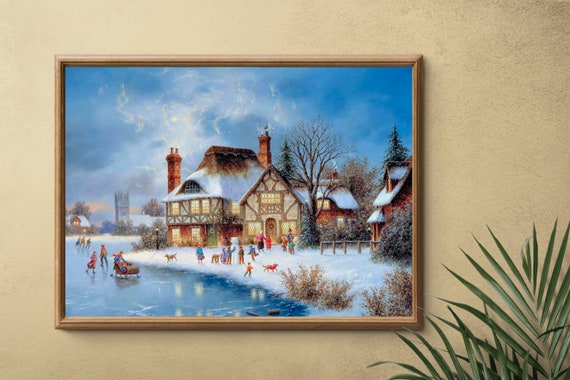The image depicts a picturesque winter scene, enclosed in a medium brown wooden frame, hung on a beige wall with the pointy leaves of a green plant visible at the bottom right corner. The scene captures an old-timey village bustling with activity on a snowy day. In the foreground, a frozen pond serves as a focal point where numerous children and adults are ice skating. Among them, a girl in a red skirt and tan shirt stands out, as does a person in a tan shirt and blue jeans. There are also people in the distance dressed in colors like orange, blue, pink, gray, red, and green, talking and playing in the snow. Specifically, some individuals are seen pushing sleds and others building a snowman. Two dogs, one brown and one reddish, are running across the snow, adding to the lively atmosphere. The village is surrounded by a mix of trees, some with green leaves and some bare, alongside bushes of different green shades. Prominent in the background is a brown house with a red façade, white snow-covered rooftops, and brick chimneys, along with other buildings, possibly including a castle. The sky is a clear blue with white clouds, contributing to the serene, festive backdrop. A brown wooden fence also lines the right side of the painting, further adding to the quaint village charm.